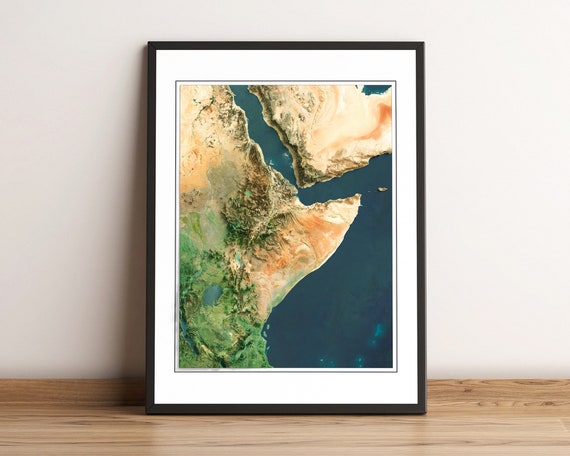This framed aerial photograph, resting on a semi-glossy wooden paneled surface and leaning against a white painted wall, exudes an earthy atmosphere. The black frame, slightly taller than it is wide, encases the photograph, which is bordered by a white mat. The positioning of the frame casts a shadow to the left, indicating light from the right.

The image captures a vast, dry landscape with minimal greenery, characterized predominantly by sandy expanses. Two landmasses are depicted, separated by a large river that opens into a bay. Notably, in the lower left-hand corner of the larger landmass, a touch of green appears around a small oasis or lake. This vividly suggests a rare pocket of life amidst the arid surroundings. The intricate detailing of the land and water, along with the thoughtful framing and ambient lighting, infuses the scene with depth and dimension.